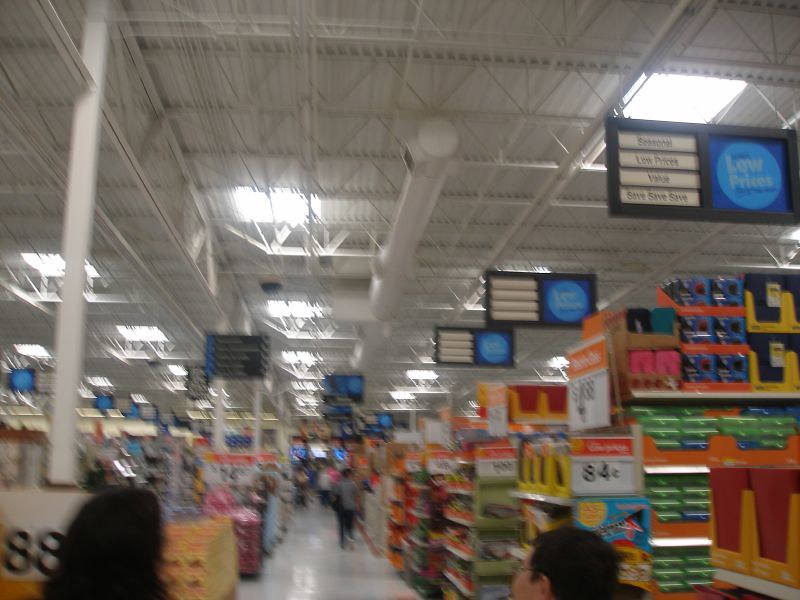The photograph showcases the interior of what appears to be a large retail store, possibly a Walmart or similar big-box store, indicated by the presence of numerous boxed items. The picture is taken from a low angle, revealing a substantial portion of the ceiling, complete with visible horizontal and vertical pipes, and several skylights. 

In the foreground, two heads can be seen: a woman with long black hair, and a boy who also has dark hair and wears glasses. The store's linoleum floor is visible and has a shiny finish. The background features multiple rows of shelves filled with merchandise, although most are too blurry to identify clearly. Some signs are hanging from the ceiling, including one that says "low prices," and another indicating items for "84 cents." A few boxes containing binders are discernible among the items on the shelves. The overall image gives a sense of the vast, organized space of the retail environment.